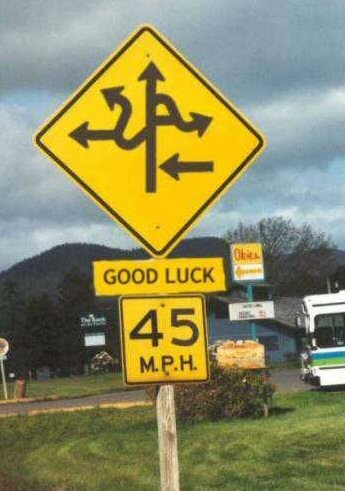This color photograph captures a prominently positioned traffic sign, set against an outdoor backdrop. The yellow, diamond-shaped sign is mounted on a wooden post at the center of the image, featuring an array of black arrows that create a labyrinthine pattern - arrows diverge and converge, with one going straight up, curvy ones twisting left and right, and several others pointing in different directions. Beneath this perplexing assembly of arrows, the sign humorously reads "GOOD LUCK" followed by a speed limit of "45 MPH." Surrounding the sign, there's lush green grass and a multitude of trees, with a hazy scene of mountains framing the distant horizon under a gloomy sky. To the right edge of the frame, a part of an RV or public bus is faintly visible. A building with unreadable marquee signage is tucked further back beyond the grasses. Additional road signs also dot the background landscape.